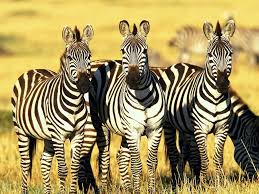In this image, three zebras stand in a close-up view, facing the camera with their distinct black and white stripes vividly displayed. Their large ears are erect, each adorned with a small tuft of black fur resembling a mohawk. One zebra, positioned to the right, appears to be sitting or lying down, its head bent as if grazing. The golden, dry grass of the African savannah stretches across the scene, blurring into the background, where the faint, indistinct shapes of additional zebras can be seen. Despite the background blur making it hard to discern details, the image captures the essence of the African landscape with muted yellows and possibly some greenery. The zebras' noses are highlighted in a deeper black or dark brown shade, enhancing their classic zebra appearance. The photograph's small size and close composition accentuate the striking presence of the zebras against the vast, dry grassland.